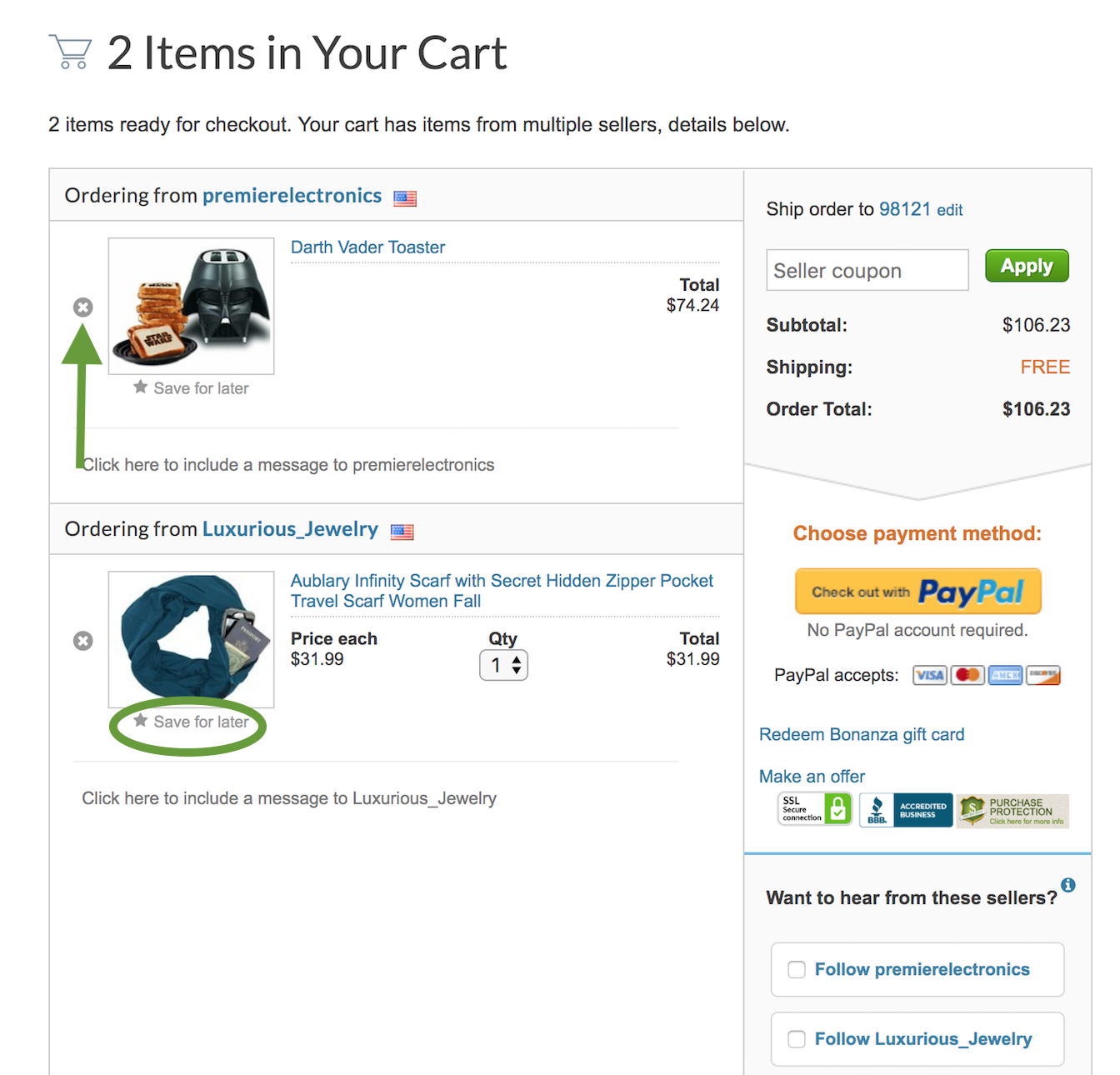The image depicts a detailed view of an online shopping cart interface. In the upper left corner, there's a small, gray shopping cart icon. To the right, there are two items currently in the cart. Directly below, a section indicates two items ready for checkout, with details showing the presence of items from multiple sellers.

Ordering from "Premier Electronics," the items listed include a Darth Vader helmet and a plate featuring either waffles or thick pieces of toast, along with a Darth Vader-themed toaster, with a combined total price of $74.24. A green arrow points up towards an "X" inside a circle above this section.

In a separate section, items from "Luxurious Jewelry" are displayed, featuring an image of an American flag and an "Aubrieri Infinity Scarf" with a hidden zipper pocket, labeled as a "Travel Scarf for Women Fall." This section also shows a blue scarf with a price of $31.99 for a single quantity. A "Save for Later" option is highlighted in green.

Further to the right, there’s a field to enter a coupon code and an "Apply" button. The subtotal for the items is $106.23, with free shipping, leading to an overall order total of $106.23. The checkout section provides an option to "Check out with PayPal" within a yellow rectangle, with PayPal accepting Visa, MasterCard, American Express, and Discover cards.